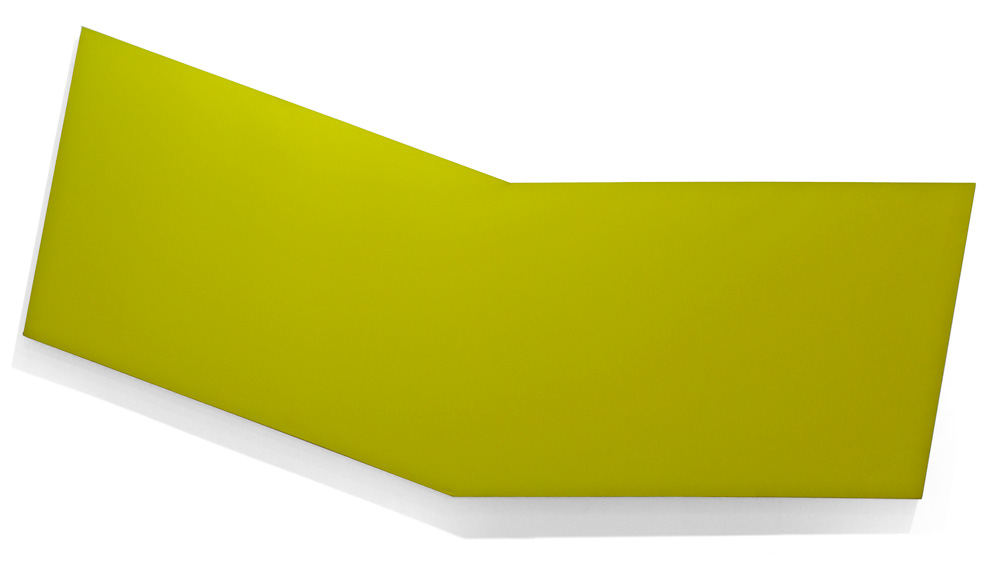The image depicts a geometric shape resembling two connected parallelograms or an open book with pages forming a 45-degree angle. It features a solid, dark yellow-green or chartreuse color, and is set against a stark white background. The color appears more intense along the edges and lighter in the center, with the left edge showing a gray-brown tint. A faint light gray shadow is cast below, adding a sense of depth. The overall shape can be interpreted as a bent stripe or a folded piece of paper, emphasizing a clean and minimalistic design.